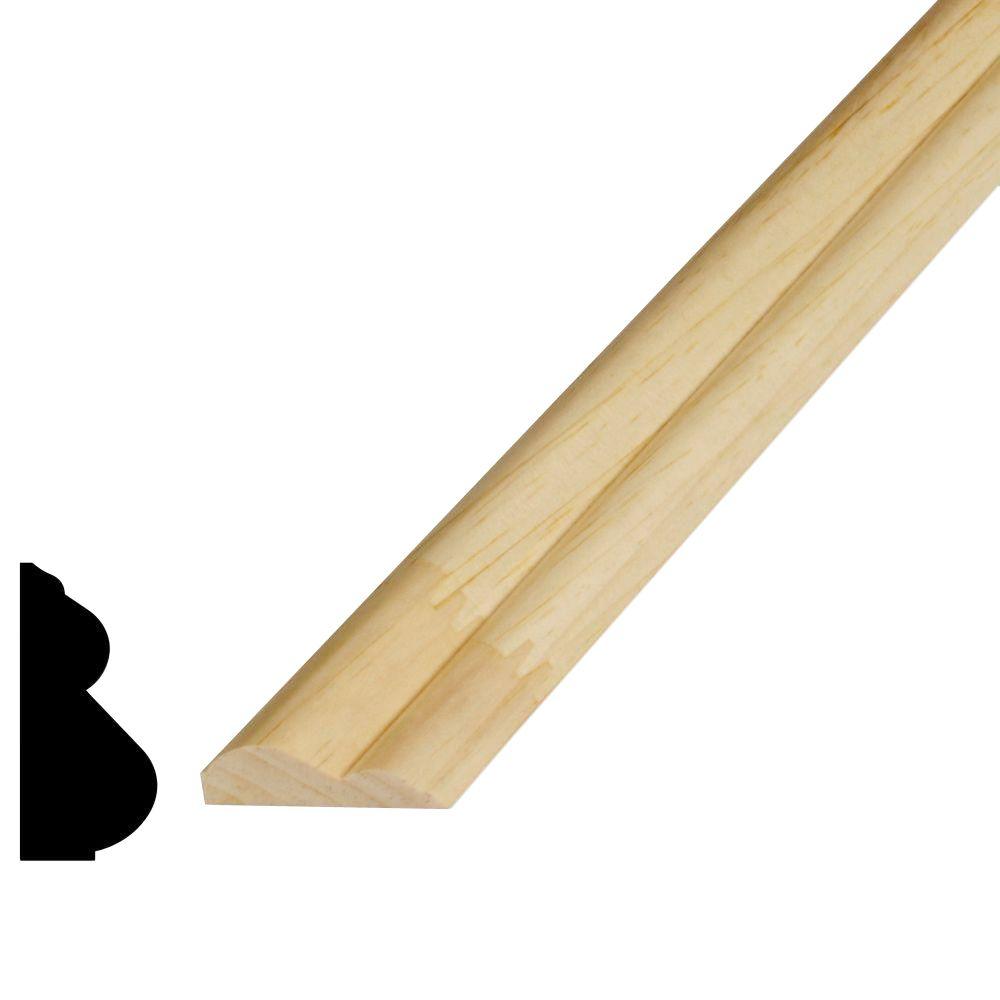In the square image with a solid white background, a piece of unfinished, natural wood trim, resembling a chair rail or floor molding, is prominently displayed. This light brown or almost flesh-colored wood, with its distinct vertical grains, stretches diagonally from the lower left corner to the upper right. The trim features a slightly beveled shape with a straight, flat cut at one end, showcasing its smooth craftsmanship. Notably, the wood includes two circular sections separated by a groove, adding to its decorative appeal. In the lower left corner of the image, there is a black outline of an irregular shape; its ambiguous form teases the viewer's curiosity, hinting it could be a symbol or an abstract figure.